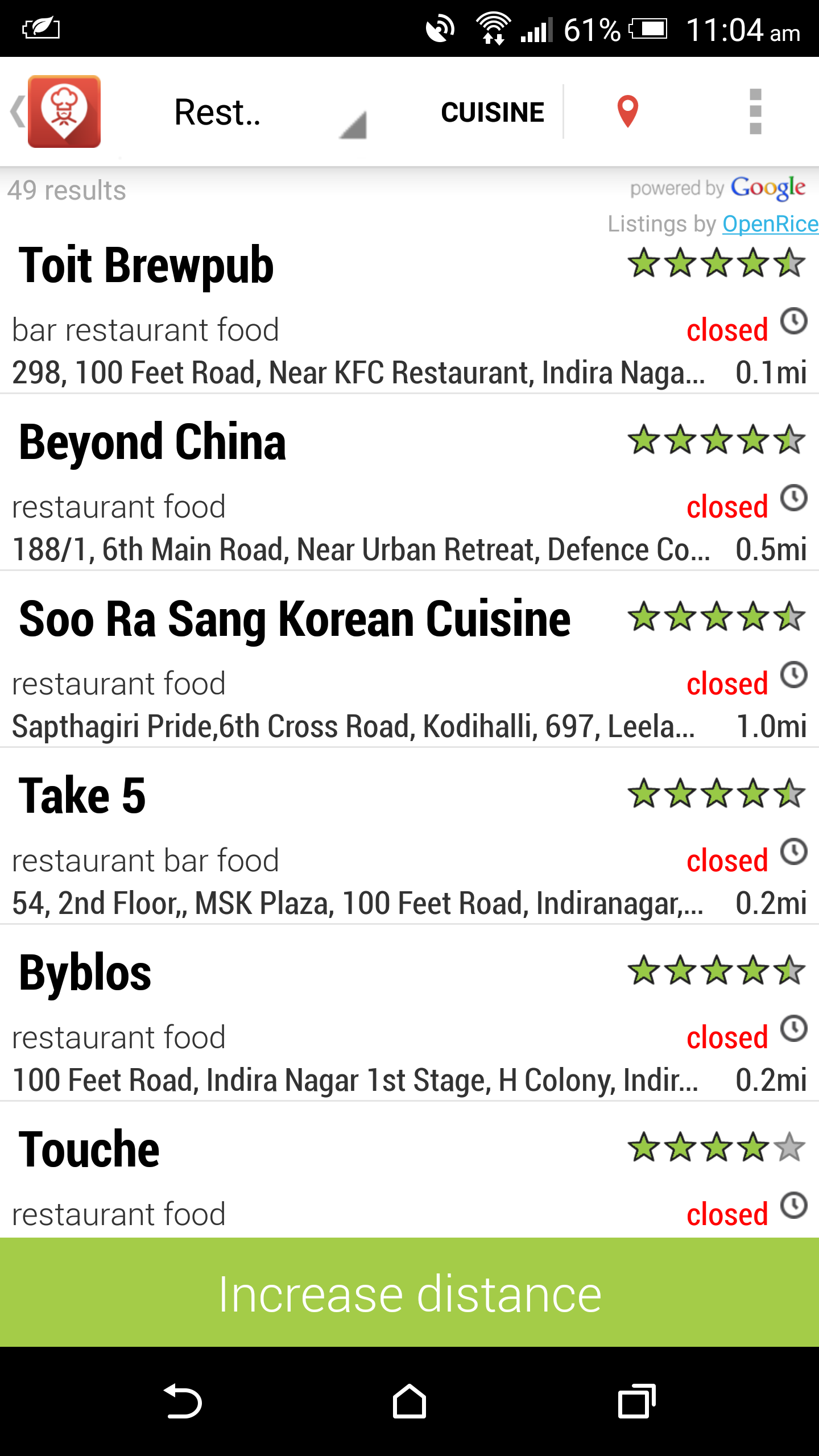In this image, we see a cell phone screen displaying a user interface for a restaurant locator application. At the top of the screen, status indicators are visible, including the connection icon, Wi-Fi signal, battery percentage (61%), and the current time (11:04 AM). Below the status bar, there are category filters labeled 'Rest,' 'Cuisine,' and a red location icon, followed by an options menu represented by three dots.

The screen shows a list of results, with "49 results" displayed at the top. Each list item contains detailed restaurant information, structured in columns. The left column shows the restaurant names in black text, with their respective locations beneath. The right column provides a 5-star rating system, the operational status (closed or open), and the distance from the user's current location.

Here are the listed restaurants:
1. **To It Brew Pub** - Closed, 0.1 miles away.
2. **Beyond China** - Closed, 0.5 miles away.
3. **Soo Ra Seng Korean Cuisine** - Closed, 1.0 mile away.
4. **Take Five** - Closed, 0.2 miles away.
5. **BYBLOS** - Closed, 0.2 miles away.
6. **Touche** - Closed, 0.2 miles away, rated 4 stars.

All listed restaurants except 'Touche' have a 5-star rating. Beneath the restaurant list, there's a green rectangle button labeled "Increase Distance." Further below, there's a black background featuring three icons.